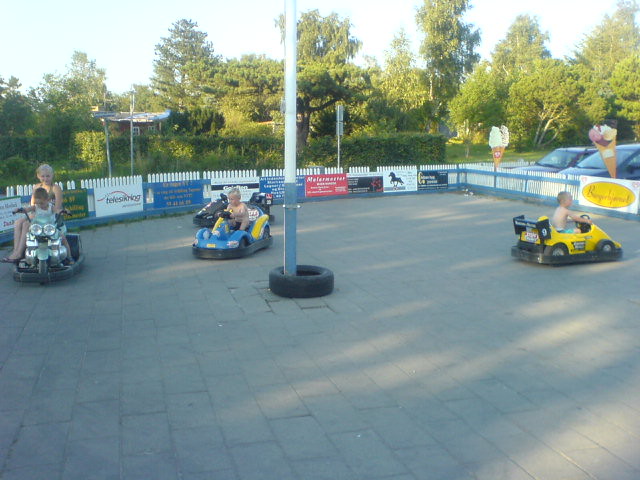The vibrant photo captures an outdoor bumper car ride station bustling with activity. Four young children are seen at the steering wheels of their small vehicles, driving around a square, fenced-off cement area with a central pole anchored by a rubber tire. To the left, a young boy is energetically maneuvering a yellow bumper car, while another boy rides alone in a blue car. A notable sight is a girl seated behind a young boy in what appears to be a motorcycle-style bumper car, distinct from the traditional cars around them. A fourth child can be spotted driving away, though the specific details of their car are less clear. The setting is bright and sunny, with a backdrop of lush shrubbery and trees, suggesting a pleasant, warm day. Surrounding the ride are white picket fences adorned with advertisements, including prominent images of ice cream cones and one featuring a horse. The cheerful ambiance suggests a family-friendly location, possibly in an Eastern European country, as hinted by some unidentifiable text on the signs.